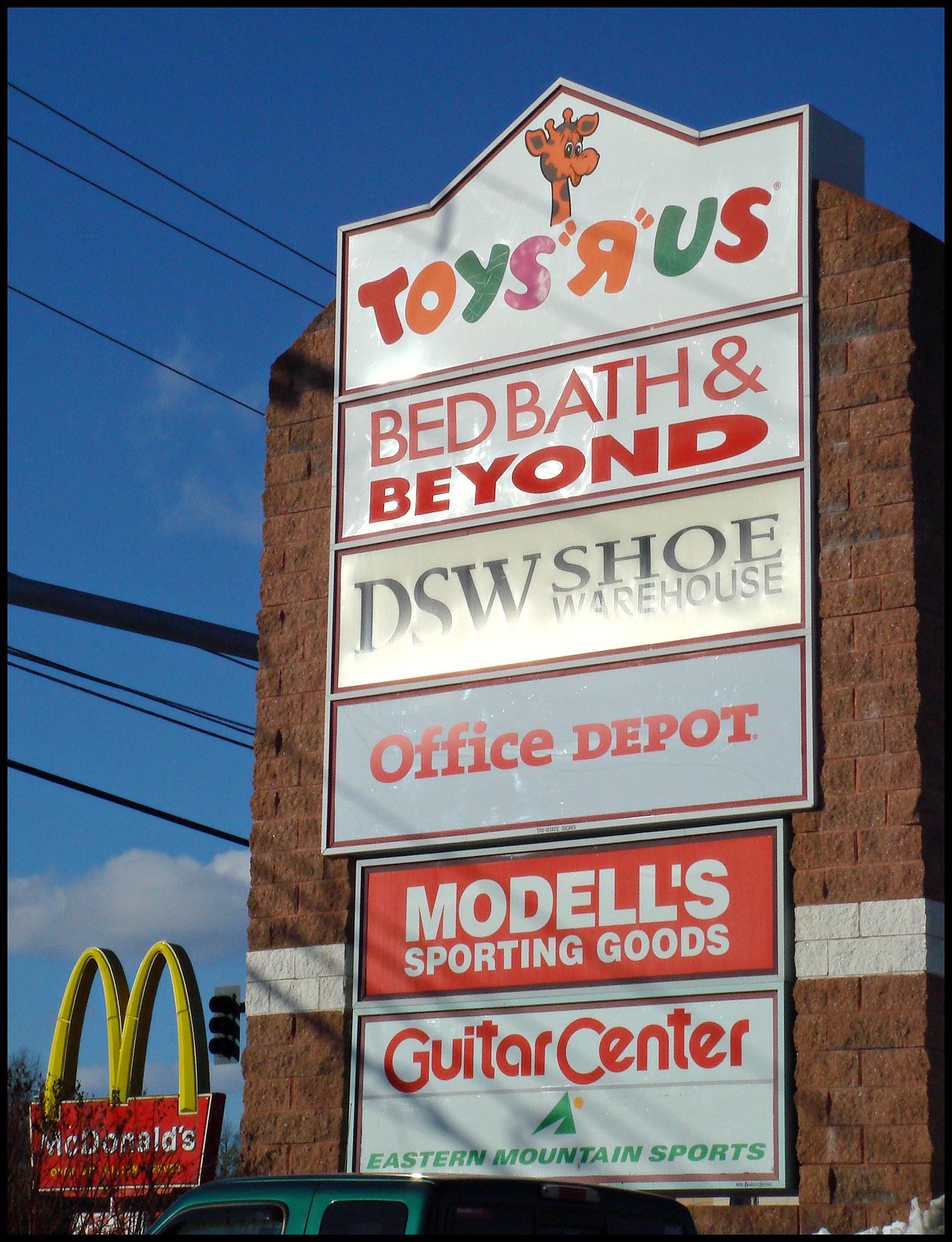The image captures an outdoor scene of a large brick-framed sign for a shopping center, prominently displaying various store logos in a vertical arrangement under a blue sky with scattered clouds. At the very top, the sign features the vibrant and colorful logo of Toys R Us, crowned with the iconic brown and black giraffe. Directly below, the sign for Bed Bath & Beyond stands out with its red lettering on a white background. Midway down, there is the DSW Shoe Warehouse branding in black on a cream background, followed by the Office Depot logo showcasing red letters on white. The sequence continues with a red sign displaying the white-lettered logo of Modell's Sporting Goods, then another white sign featuring the red-lettered Guitar Center logo. Just below this, the logo for Eastern Mountain Sports appears in green. The scene includes additional elements such as power lines stretching off to the left and a glimpse of a green car's roof at the very bottom. In the bottom-left corner, partially visible, is a McDonald's sign with its famous Golden Arches on a red background.